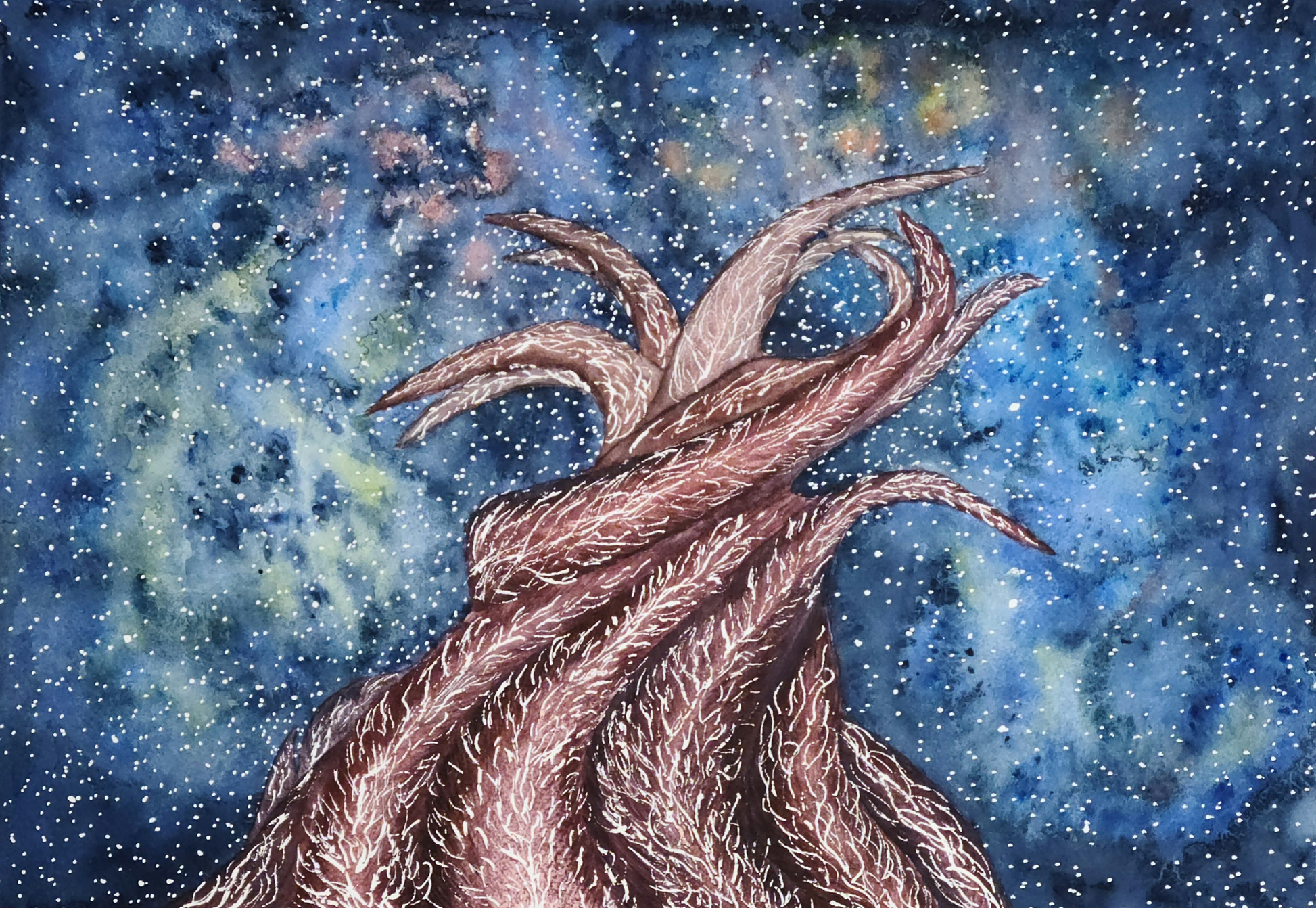The image depicts an abstract graphic painting of a tree immersed in a cosmic or celestial setting, giving the impression of a fantastical scene possibly set in space. The tree's branches are intricately tangled and pointed, colored primarily in dark brown with prominent white markings or veins. The unique background transitions from a deep black and dark blue at the edges to lighter shades of blue towards the center, dotted with white specks that evoke the feeling of stars or heavy snowfall. Additional hues in the background include peach-rose on the top left, yellow on the top right, and a greenish tint near the center left. These colors blend seamlessly with the various blotches and clouds of whitish-gray, giving the image an ethereal and otherworldly quality. The combination of these elements creates a mystical visualization where the tree, with its lighter central tendril, stands out strikingly against the celestial backdrop.